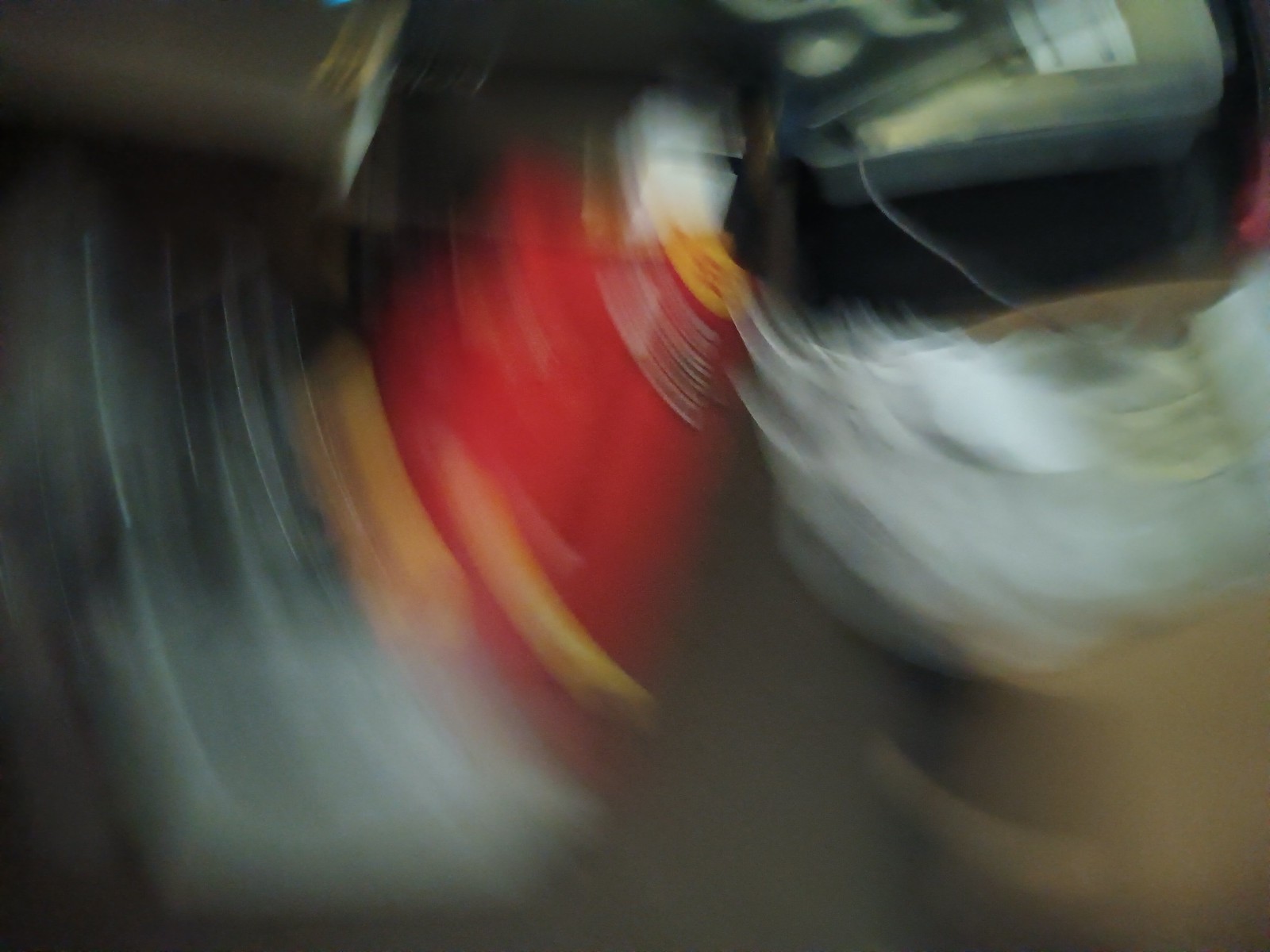In this extremely blurry image, a predominantly light gray color occupies the bottom portion, extending to the left-hand side. Above this, a patch of yellow appears, transitioning into a bright red section. Moving upward, gray lines emerge, culminating in a cube-like gray object. The top left corner features a dark gray hue, while the top right showcases an indistinct object in black and yellowish gray. Below this area, a series of white colors unfolds, leading to a light brown section in the bottom right corner. The severe blurriness of the image renders only these colors discernible.